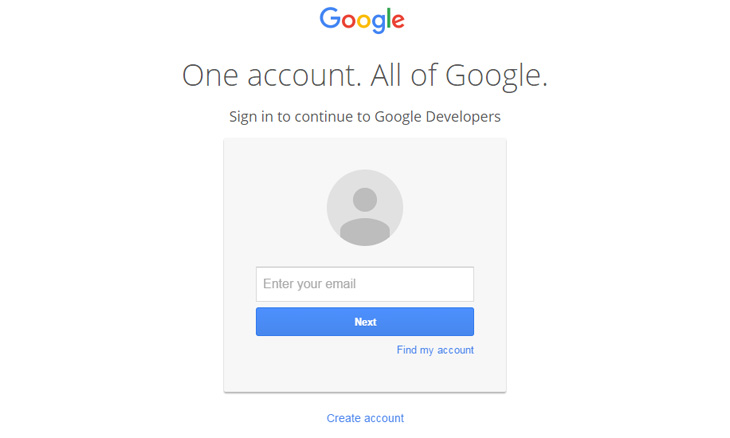The image depicts the Google login page tailored for developers. At the top of the page is the iconic Google logo. Just below it, there is a statement in black lettering against a white background that reads "One account. All of Google." Beneath this, smaller text states "Sign in to continue to Google Developers." Lower down is a light gray box containing an entry field with a placeholder for an email address, accompanied by a small gray circle featuring a generic human avatar. Adjacent to this entry field is a blue button with "Next" written on it in white text. To the bottom right of this button, there is a clickable text link in blue that reads "Find my account." Just outside the gray box, at the bottom, is another blue text link that says "Create account." This entire setup indicates that the page is specifically intended for developer login access to Google Developer services.